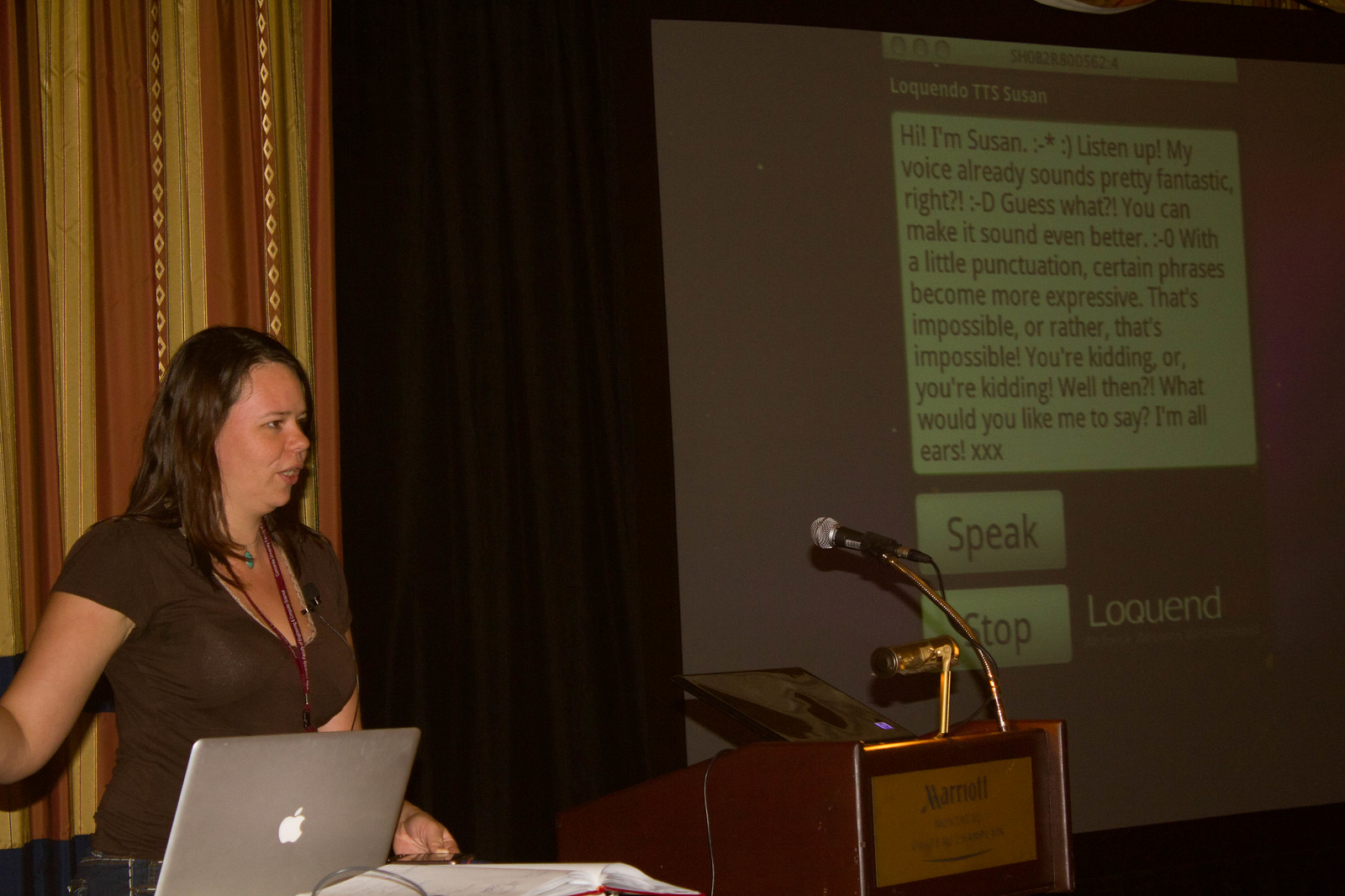In this photograph, positioned in the lower left-hand corner, there's a curvy woman with long brown hair, wearing a short-sleeved, low-cut brown shirt with a red lanyard around her neck. She appears to be speaking, as her mouth is slightly open. She stands at a wooden lectern featuring two microphones and the word "Marriott" in gold lettering. In front of her, off to the side, there is a silver MacBook and some papers. The background consists of brown and gold curtains, and to her right, there's a large projection screen. The screen displays a text message that reads, "Hi, I'm Susan. Listen up. My voice already sounds pretty fantastic, right? Guess what! You can make it sound even better. With a little punctuation, certain phrases become more expressive. That's impossible! Or rather, 'that's impossible?' You're kidding. Or, 'you're kidding? Well then, what would you like me to say? I'm all ears." The screen also shows buttons labeled "speak" and "stop," along with the logo for "Loquend." The scene primarily focuses on her as she delivers a speech.